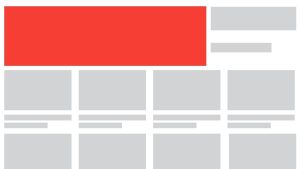The image displays a minimalist design composed of various geometric shapes set against a pristine white background. Dominating the top left corner, there is a large red rectangle, which is the most prominent shape. Adjacent to this, on the right, is a smaller gray rectangle with an even smaller gray rectangle positioned directly beneath it. Further down, the design features two horizontal rows, each comprising four evenly spaced gray squares. Nestled between these two rows are two very small gray rectangles, with the upper rectangle being slightly longer than the lower one. The crisp white negative space around and between the shapes adds to the clean and modern aesthetic of the composition.